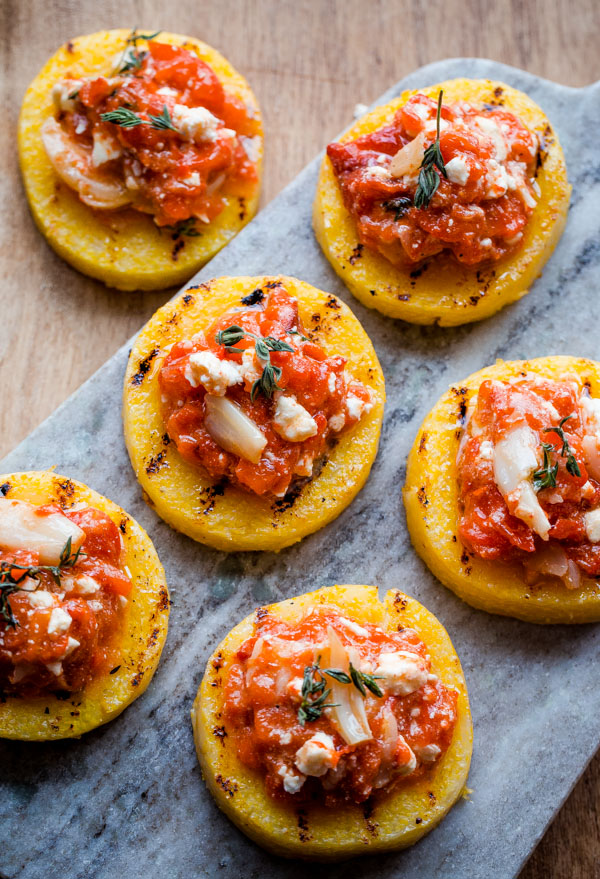The image captures a rustic and appetizing food presentation that appears straight out of a recipe book. Six small, circular food items, resembling grilled pineapple slices, are topped with a vibrant red sauce, chunks of mozzarella or goat cheese, and a sprinkle of greenery, possibly herbs. Five of the pieces rest on a gray marble or granite serving board that features a mix of gray and black shades, while the sixth piece is placed directly on a rustic brown wood table adjacent to the serving board. Each piece exhibits visible grill marks, suggesting they have been grilled to perfection. The composition of the items—five on the board and one on the table—creates an inviting and rich visual presentation, possibly of a crostini or bruschetta-style appetizer.